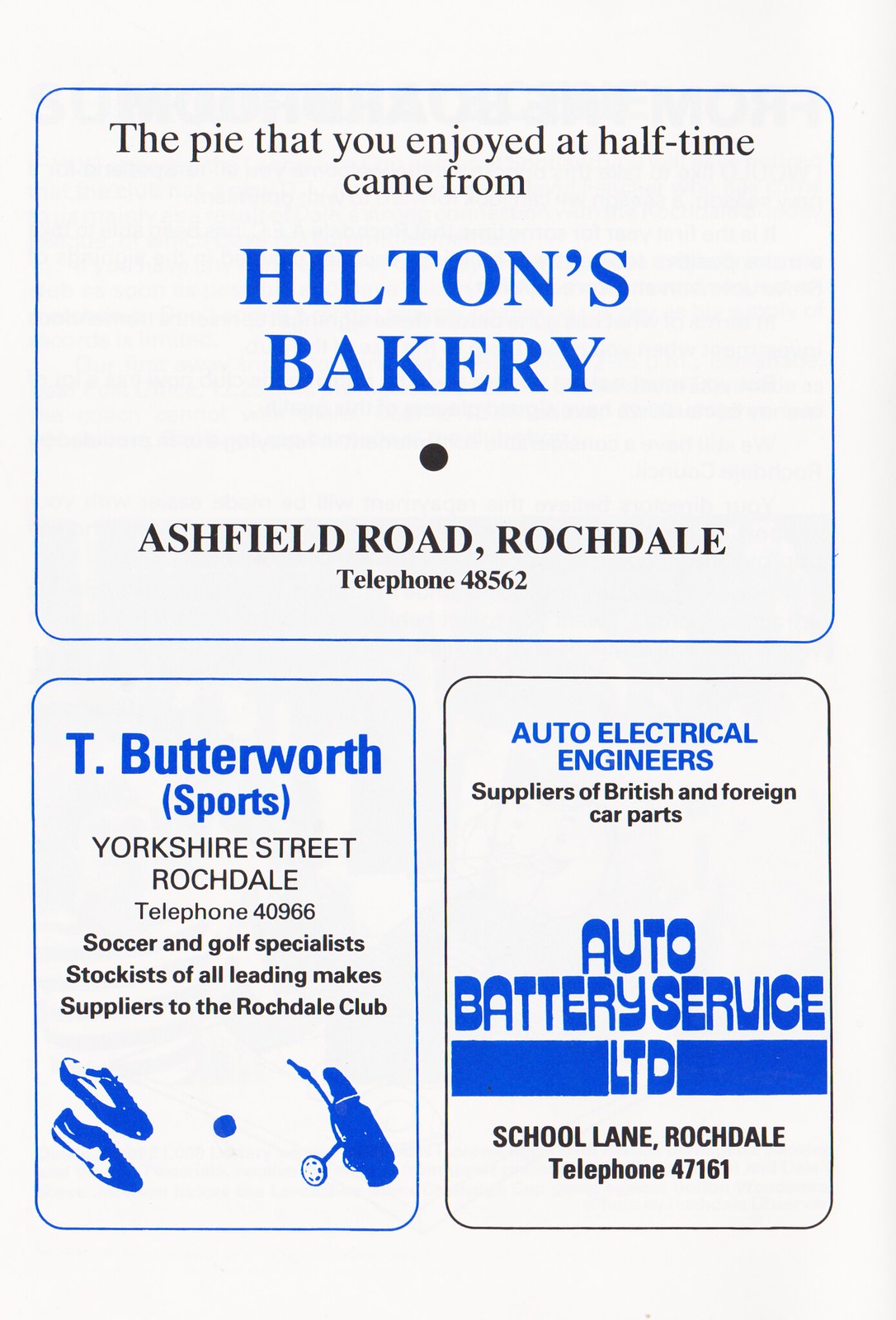This image is a page of advertisements from a game day program, likely for a soccer game in Rochdale, featuring three distinct ads. The top half is dominated by a large, rounded blue square with black and blue text, advertising Hilton's Bakery. It notes, "The pie that you enjoyed at halftime came from Hilton's Bakery," located on Ashfield Road, Rochdale, with a telephone number of 48562. The bottom left section contains a blue square promoting T. Butterworth Sports, located on Yorkshire Street, Rochdale. The advertisement highlights that they are soccer and golf specialists and stockists of all leading makes, supplying the Rochdale Club, with a telephone number of 4966. Illustrations of two shoes and a golf caddy in blue are also present. The bottom right ad is for Auto Battery Service Limited, framed in a black square with blue and black text. It describes the company as auto electrical engineers and suppliers of British and foreign car parts, situated on School Lane, Rochdale with a telephone number of 47161.